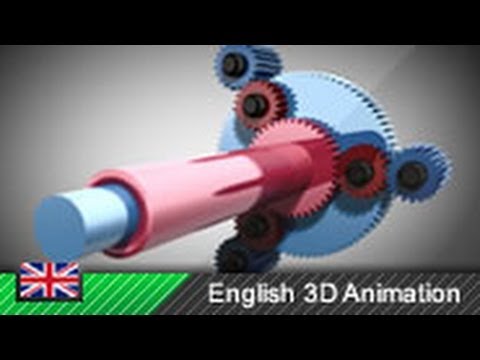The paused video depicts a detailed 3D animation described as "English 3D animation" in white font at the lower right-hand side of the screen. Prominently, the British flag, characterized by a red cross, a lighter red X, a white X, and shaded blue sections, is displayed in the bottom left corner. At the bottom of the screen, a bar with diagonal lines, half filled with green, possibly acting as a loading indicator, accentuates the visual. 

The animation showcases a complex gear mechanism on a pale gray background. Central to the graphic is a large blue gear with three smaller attached red and blue gears. A long pale blue shaft is encased in a red holder, which is connected to the main red gear. This primary red gear interacts with three additional smaller red gears on its top. These smaller gears, in turn, spin three smaller gray gears positioned on the outside, which drive the large central gray gear on the bottom. The overall composition features two thick black bands at the top and bottom, framing the scene.